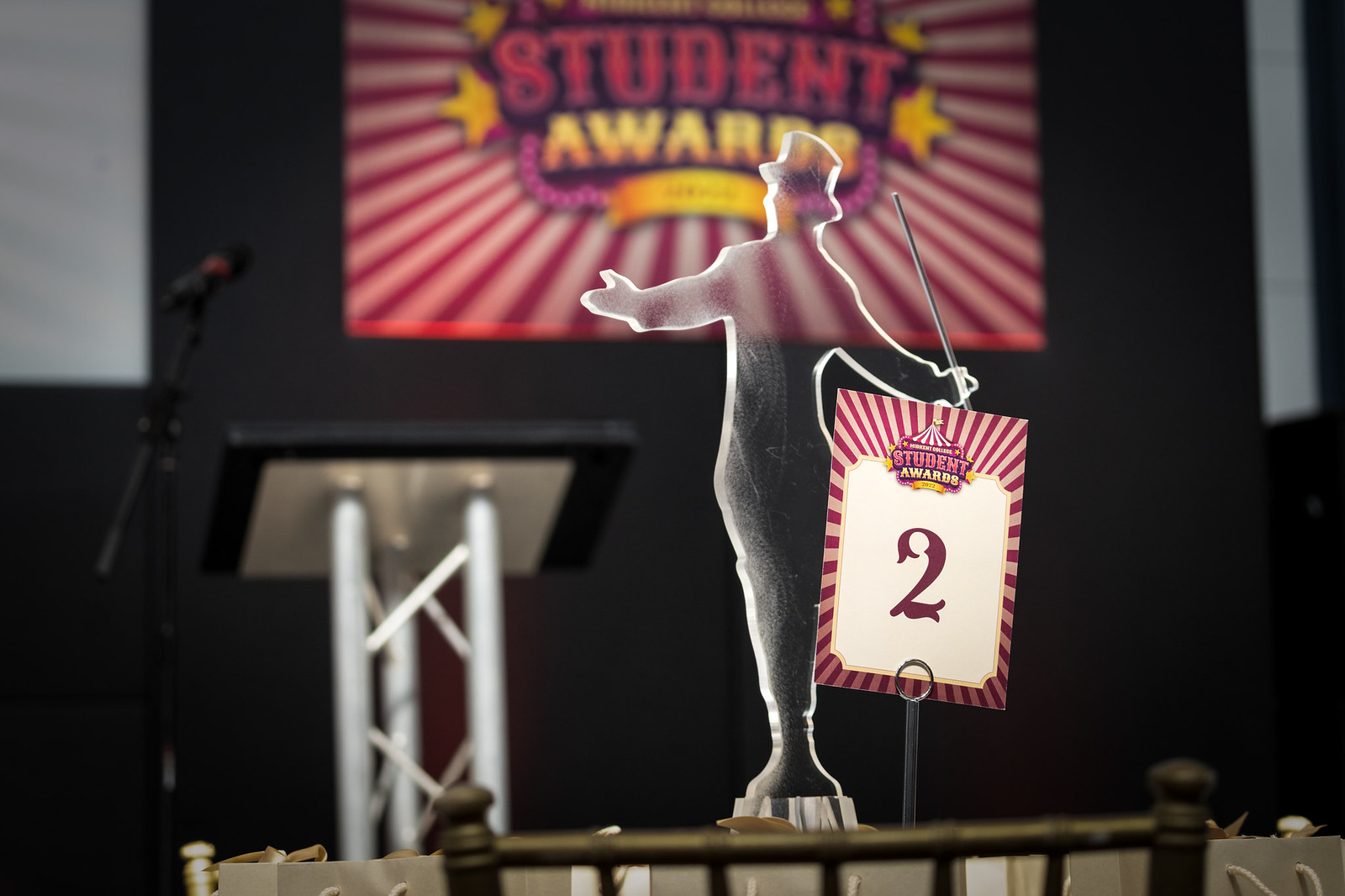The photo depicts an indoor award ceremony setup for student award winners. Dominating the background is a vibrant sign that reads "Student Awards," illuminated by rays of white and red light. In the foreground, there is a meticulously set table featuring a prominent statuette, which is either plastic or glass and is notably translucent. The statuette depicts a figure wearing a top hat, with an elongated baton in its right hand and an outstretched left hand. Beside it, a placard reads "Take Number Two." Adjacent to the table stands a podium fitted with a microphone, awaiting the forthcoming announcements or speeches.